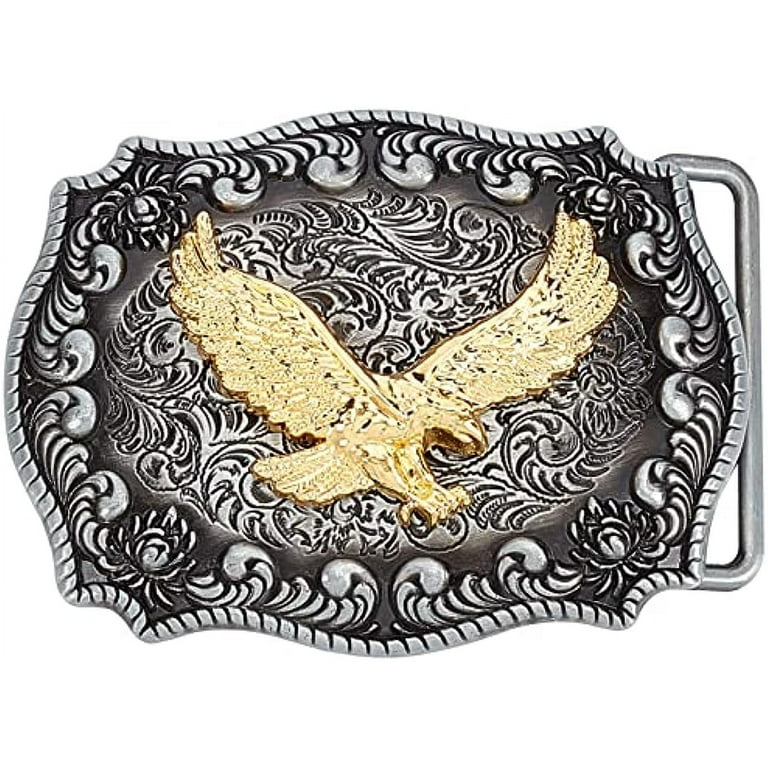The image depicts a highly ornate belt buckle made from a silvery metal with dark spots, suggesting it might be iron. The overall shape of the buckle is near-rectangular with rounded edges. Intricate decorative elements include a detailed rope-like pattern around the perimeter and various wavy, leaf-like, and floral designs adorning the central area. Dominating the center is a striking bronze or gold eagle, poised mid-swoop with wings spread wide as though about to capture something. The background behind the eagle is silver, enhancing its prominence. To the right of the buckle is a slot designed to allow a belt to slide through and secure it in place. The buckle is set against a plain white background, emphasizing its elaborate artistry and craftsmanship.